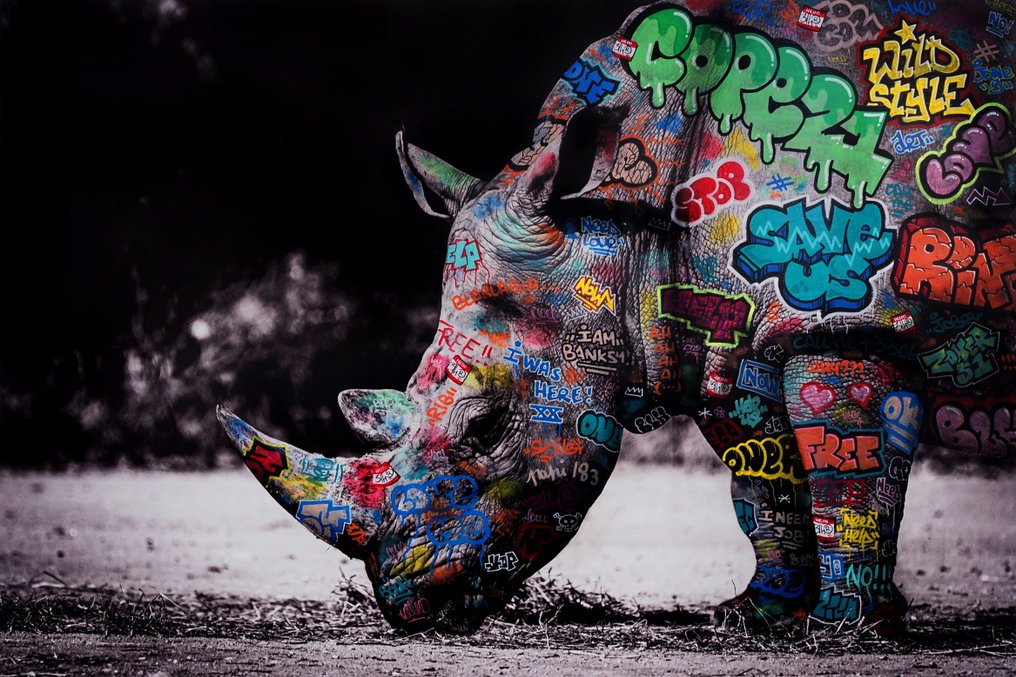This captivating image encapsulates the powerful juxtaposition of nature and urban art. The main focus is a rhino, its head lowered as if grazing on a hidden patch of hay. The photograph is mostly monochromatic, with the background shrouded in deep black, further accentuating the intricate graffiti adorning the rhino’s body. The graffiti, colorful and vibrant, transforms the gray silhouette of the rhino into a dynamic canvas of urban expression.

Prominent graffiti elements include: 
- The phrase “C-O-P, P-21” in green near the top of its body.
- “Wild Style” splashed in bold yellow.
- On the rhino’s shoulder, the plea “Save Us” is scrawled in blue, juxtaposed with the letters “R-I-N” in red nearby.
- The word “Free” appears prominently in red across the top of its leg, accompanied by two delicate pink hearts.
- On the cheek, the cryptic proclamation “I am Bank 54” stands out.
- The messages “I was here” in blue and “Free” on its forehead signify human presence and intervention.

The contrasts between the rhino’s natural form and the vivid, rebellious strokes of graffiti paint create a poignant and thought-provoking visual narrative, asking viewers to ponder the impact of human actions on wildlife and nature.